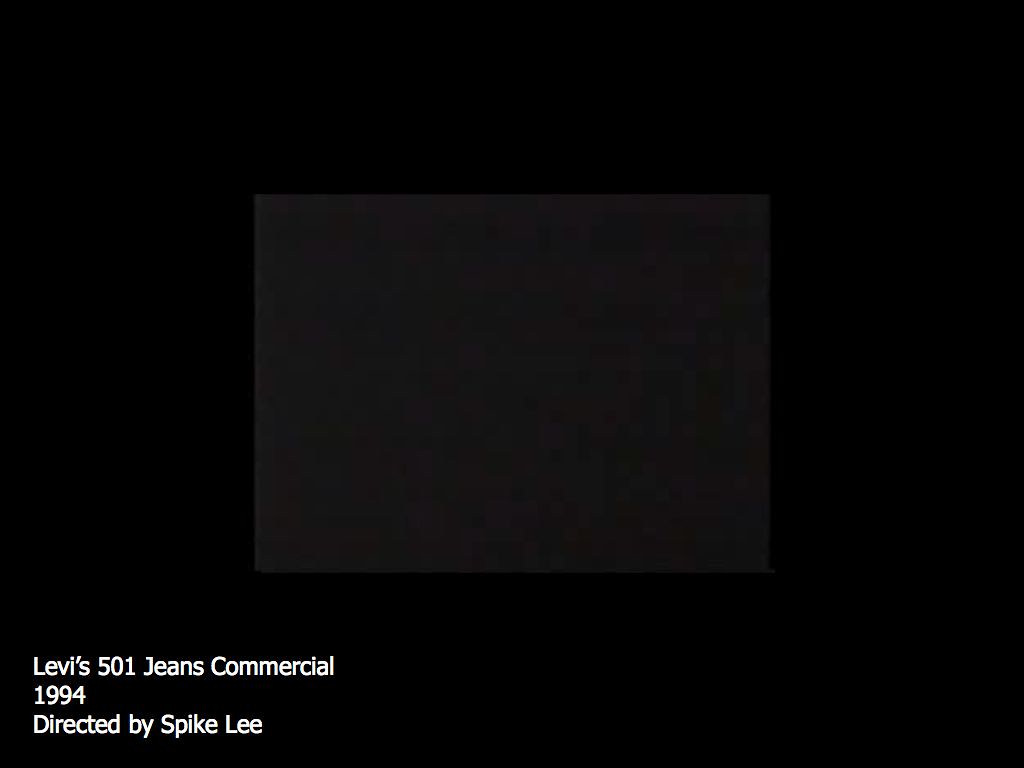The image depicts a digital screen grab, likely the initial frame of a video commercial. The background of the image is completely black, creating a stark contrast with a smaller, centrally-located rectangle. This inner rectangle, slightly pixelated and rendered in various shades of gray, along with hints of greens and blues, appears to be the starting frame where the video content is supposed to begin. Adding context, the bottom left corner of the image displays white text providing crucial information: "Levi's 501 Jeans Commercial, 1994, directed by Spike Lee." This text is arranged in three lines and indicates that the screenshot captures the opening moment of a 1994 commercial directed by Spike Lee, potentially sourced from a YouTube video or similar platform.